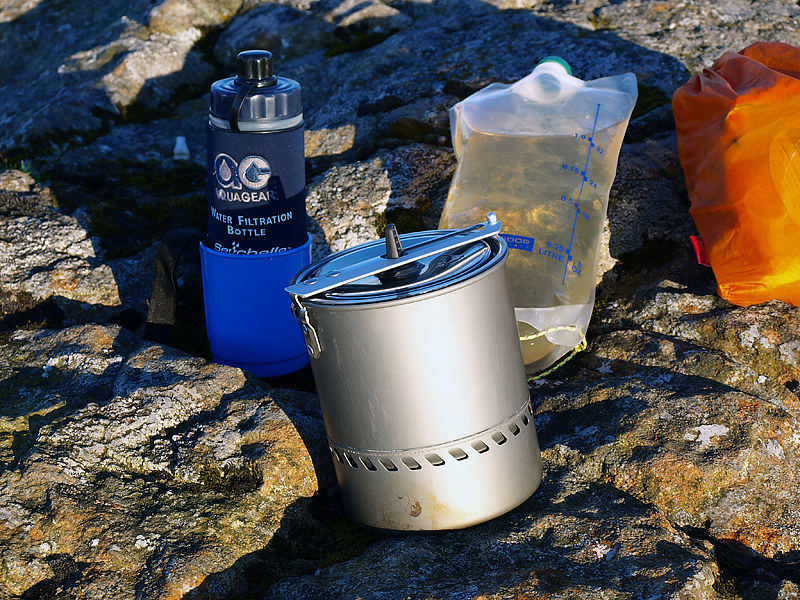In this photograph taken during the early morning or late evening, a collection of camping gear is artfully arranged on a rugged, speckled rocky surface with hues of dark gray, light gray, and occasional gold flecks. Dominating the center of the image is a large, non-reflective metal pot with a secure clasp lid, possibly used for boiling or purifying water. To its left, a light blue plastic cup contains a dark blue, velvety AquaGear water filtration bottle, the cozy around it marked with the brand name and two symbols, and topped with a nozzle. On the right side of the pot, there's a tall, clear plastic bag filled with a murky brown liquid, possibly water. Towards the top left corner of the photograph, an orange plastic bag, potentially a type of backpack, sits partially open, its contents indistinguishable. The entire scene is bathed in low-angle sunlight, casting defined shadows over the objects, highlighting their textures and emphasizing the natural beauty of the weathered rock beneath them.